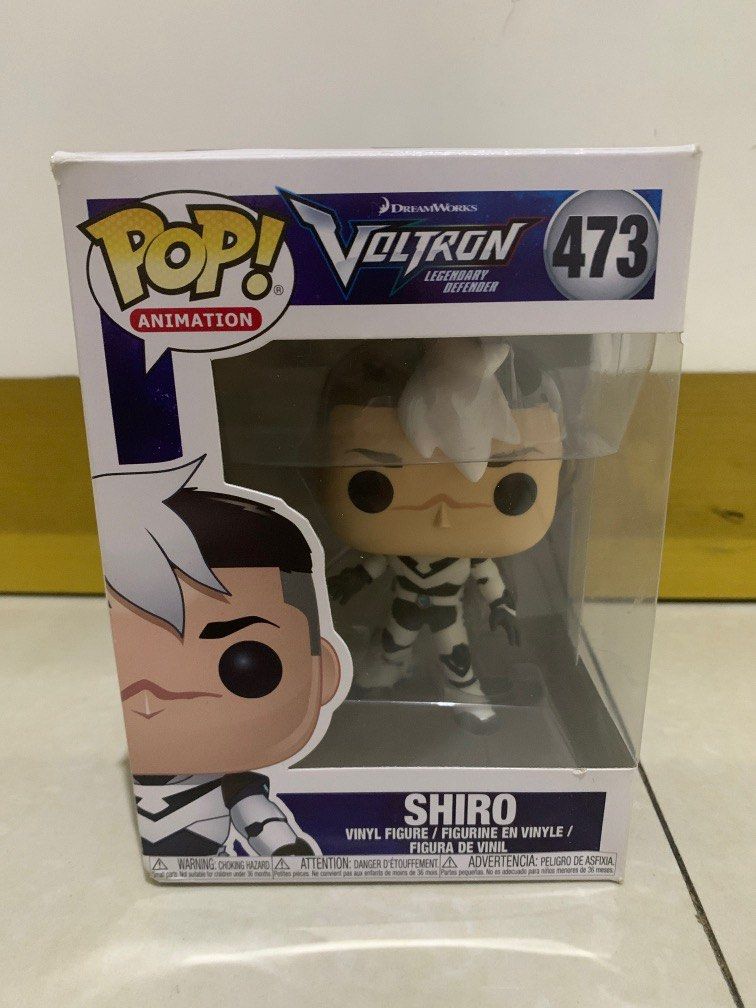This is a detailed photograph of a Funko POP Animation vinyl figure, featuring the character Shiro from DreamWorks' "Voltron: Legendary Defender." The figure is securely enclosed in a cube-shaped cardboard box with a clear plastic window on the front and side, allowing a full view of the collectible inside. 

The top of the box prominently displays the "POP Animation" label in yellow letters with "animation" in red within a speech bubble. Below this, "Voltron 473" is written, indicating the series. The name "Shiro" is printed in large letters, accompanied by translations in multiple languages, emphasizing its international appeal.

Shiro, wearing a black and white jumpsuit with alternating hues, stands with his left foot slightly forward. His character design features a notably large head with stark contrasts: black hair at the back and a distinctive white streak running through the middle. His light-skinned face bears a scar across the nose, and the typical Funko POP aesthetic gives him exaggerated, large black eyes. The box also includes safety information, warning of a choking hazard. Set on a tile floor, this collectible remains pristine and unopened, ideal for any fan or collector.